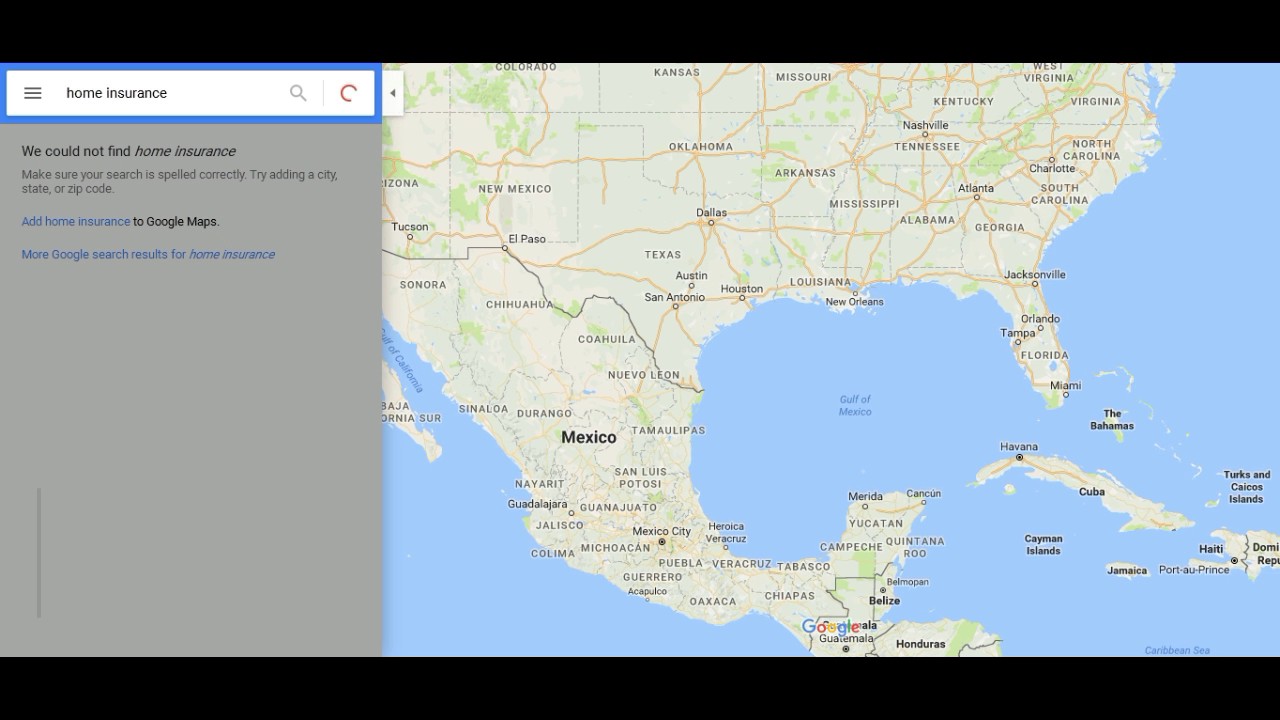This image appears to be a screenshot from a computer. The screen is bordered by black bands at both the top and bottom edges. The left side features a gray background with a prominent white search bar at the very top, encased in a blue rectangle. Inside the search bar, which shows three small vertical lines to the left, the phrase "home insurance" is typed. Below the search bar, the gray background extends down with a message stating, "We could not find home insurance. Make sure your search is spelled correctly. Try adding a city, state, or zip code." The message also offers the option, "Add home insurance to Google Maps," with "Add home insurance" appearing in blue text. An additional suggestion reads, "More Google search results for home insurance." 

To the right of this search area is a map showing the United States at the top and Mexico at the bottom, with the Gulf of Mexico visible to the right. The rest of the image to the right of the search results and below the message on the left side is largely blank gray space.